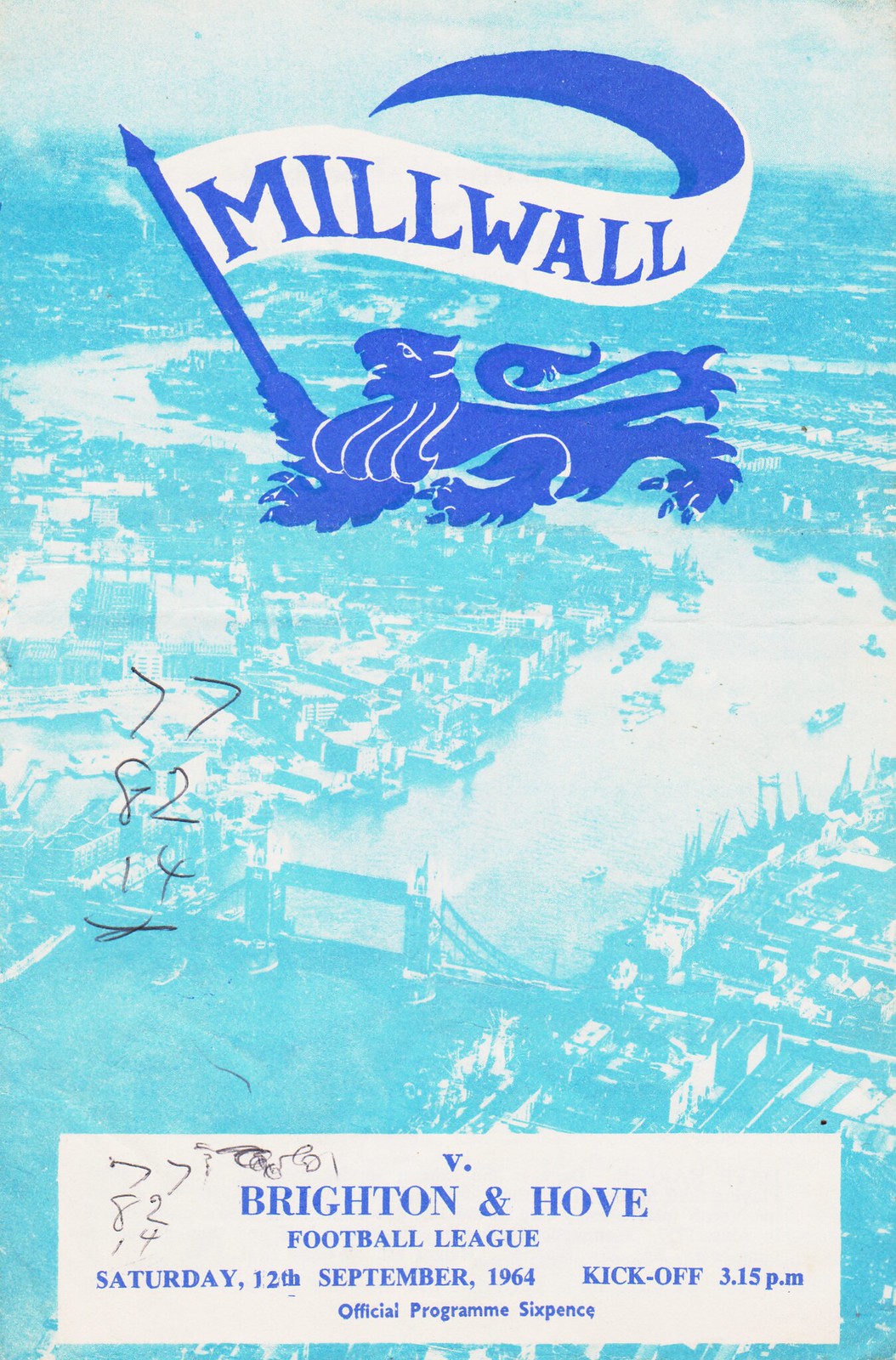This image is an official program cover for a soccer event, specifically a match between Millwall and Brighton & Hove Football League, held on Saturday, 12th September 1964, with a kickoff at 3.15 p.m., and it cost sixpence. The top of the cover features a dark blue emblem of a lion facing left, holding a flagpole with a triangular flag. The banner on the flag reads "Millwall" in bold letters. Behind the lion, there is a background illustration in a faded bluish tint depicting a river, possibly the Thames, winding through a cityscape that includes the London Bridge and surrounding buildings. 

On the left side of the cover, there is handwritten notation with the numbers "77," "82," and "14" stacked vertically, repeated in another spot on the cover. Additionally, there is a small black squirrel lying below the numbers. The bottom of the cover also features a white rectangular box containing the text "V. Brighton & Hove Football League" alongside the date and time details. The entire image has a vintage, slightly washed-out bluish appearance, giving it an old-timey feel.